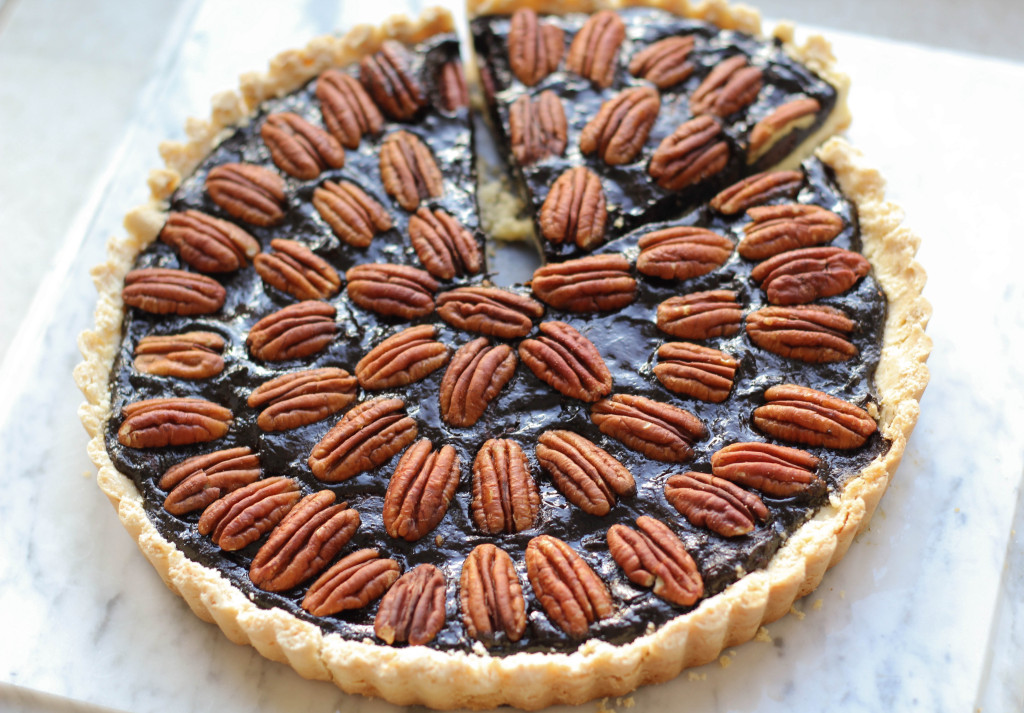This image showcases a mouthwatering chocolate pecan tart, meticulously presented on a marble countertop or cutting board, slightly out of focus to emphasize the dessert's allure. The tart features a beautifully arranged spiral pattern of pecans atop a rich, dark chocolate filling. The traditional wavy crust, hinting at its homemade origin, is a light golden brown and slightly flaky. One slice towards the right has been carefully cut but remains within the tart, revealing some crumbs and highlighting the tart's approximate half-inch thickness. This delectable tart, likely yielding about six servings, exudes an irresistible richness, perfectly staged for a baking showcase.